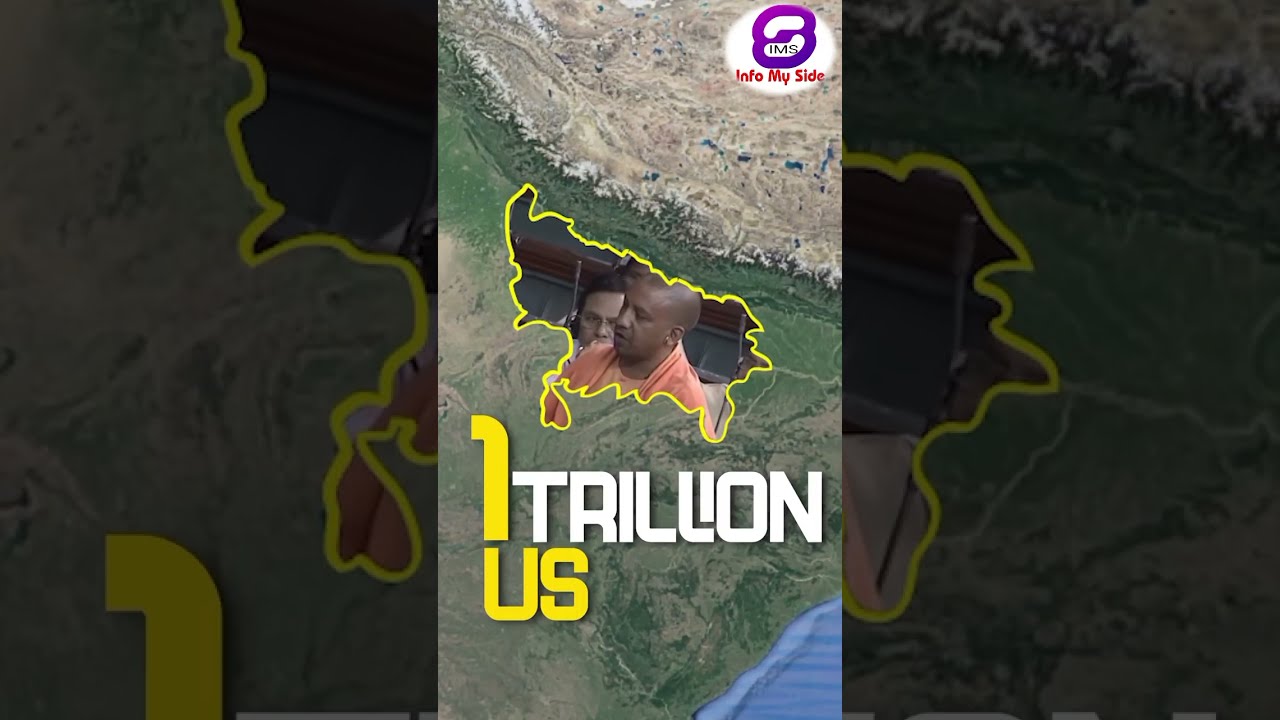The image is a horizontal rectangular graphic divided into three segments. The outer segments on the left and right sides are large, darkened areas with a low exposure, featuring a mostly browned-out appearance. These flanking sections serve to highlight the center frame, which is clearer and reveals a detailed map-like image.

The central frame showcases an aerial or satellite view of a landmass, possibly representing an unidentified country. The landscape's lower region is predominantly green, suggesting fields or vegetation, while the upper region transitions into brown, hinting at mountainous terrain. Superimposed on this terrain is a more specific depiction of the landmass, prominently outlined and backed by contrasting colors for clarity.

In the heart of this central map, two people can be seen, including a black man wearing an orange shirt, which adds a human element to the geographical focus. Furthermore, near the bottom of the central frame, bold text is displayed in two lines: the top line reads "one trillion" in white, and the bottom line reads "U.S." in yellow. Also notable is a small blue diagonal segment in the lower right corner, suggesting a body of water, and a beige diagonal portion extending from the green vegetation into the top right corner.

Above the text in the central portion, there’s mention of an "info on my side" and a noticeable IMS trademark or copyright symbol, adding a layer of informational detail and authenticity. The entire image presents a multifaceted map with embedded human and textual elements, creating a mosaic of geographical and contextual information.